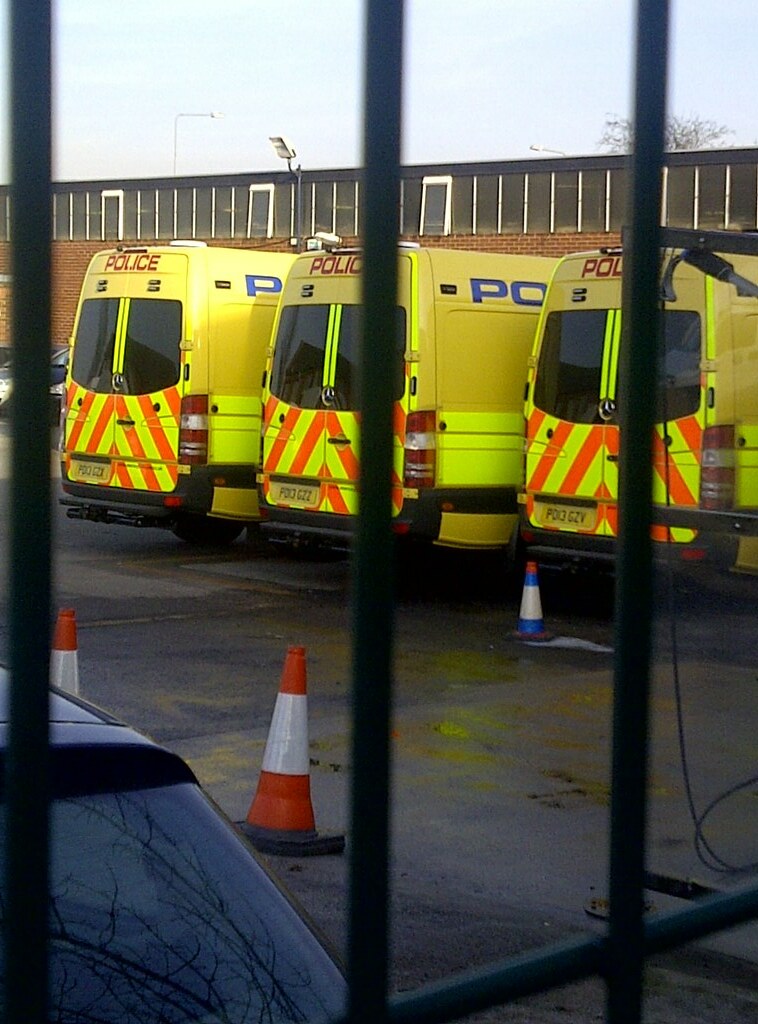This photo captures a scene taken outdoors through a sturdy iron gate with vertical bars, depicting a parking lot of a police station in a foreign country, likely in Europe. Dominating the image are three striking bright yellow police vans, each accented with fluorescent yellow and orange hazard stripes on their lower sections. The back doors prominently display "POLICE" in large red letters above two darkly tinted black windows. In large blue font, the word "POLICE" is also inscribed on the sides of these vehicles. The license plates, which all start with "PO" and end in "GZ", are long, skinny, and yellow, emphasizing their non-American origin. 

Scattered throughout the scene are several traffic cones: two orange with white stripes, one with an orange top adorned with blue and white colors, and an additional blue cone further back. A partially visible black car is noticeable in the lower left-hand corner of the image, adding to the sense of depth. The lot's surface appears to be dark asphalt or cement, wet from recent weather.

In the background stands a tall brick building with numerous windows at its top, and partially obscured by the structure is a tree extending into the clear, light blue sky. Some cables hang down from an indeterminate source, adding a chaotic element to the otherwise orderly scene. The photograph, rich in detail, reveals an environment that combines the austere functionality of a police station with the subtleties of its foreign setting.